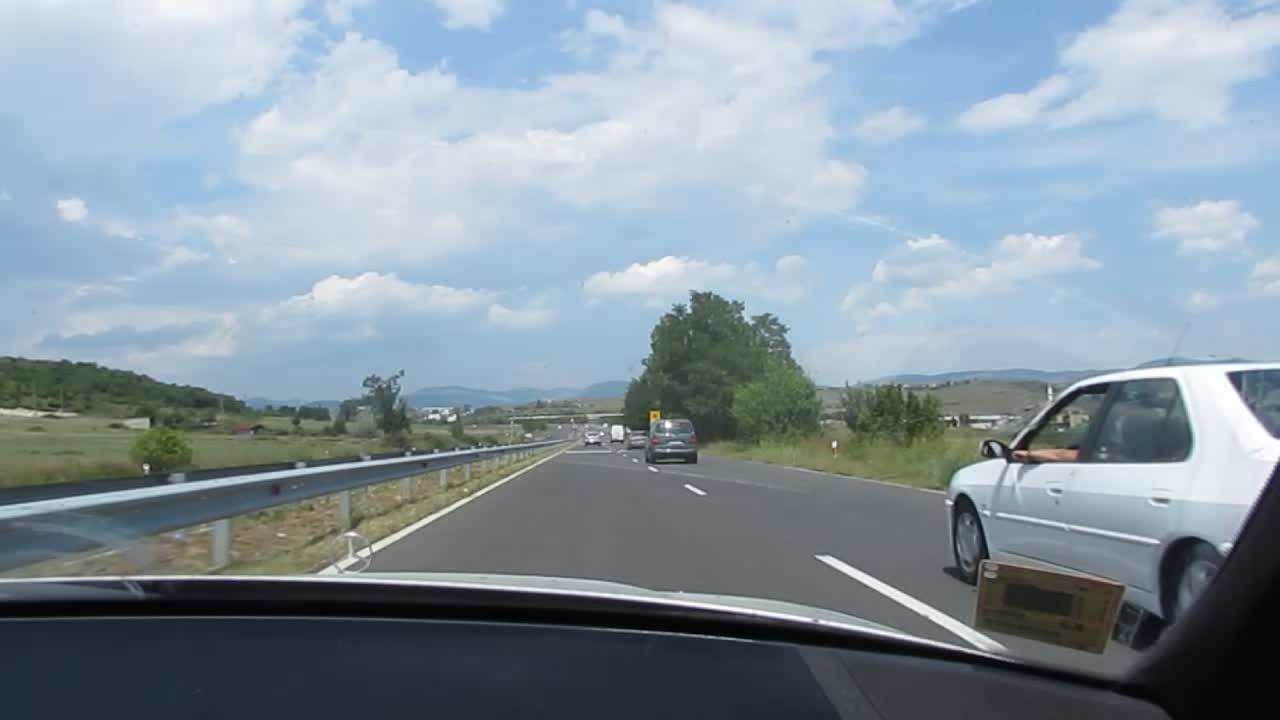Captured from the passenger side of a vehicle, this image provides a perspective through the windshield. The dashboard spans across the frame from left to right, and part of the interior structure that holds the windshield is visible on the lower right-hand side. An inspection sticker is affixed to the windshield in the lower right corner. The car is positioned in the second lane of a two-lane road. Ahead, in the first lane to the right, a white car is visible. Additionally, several other vehicles can be seen on the road, contributing to a typical traffic scene.